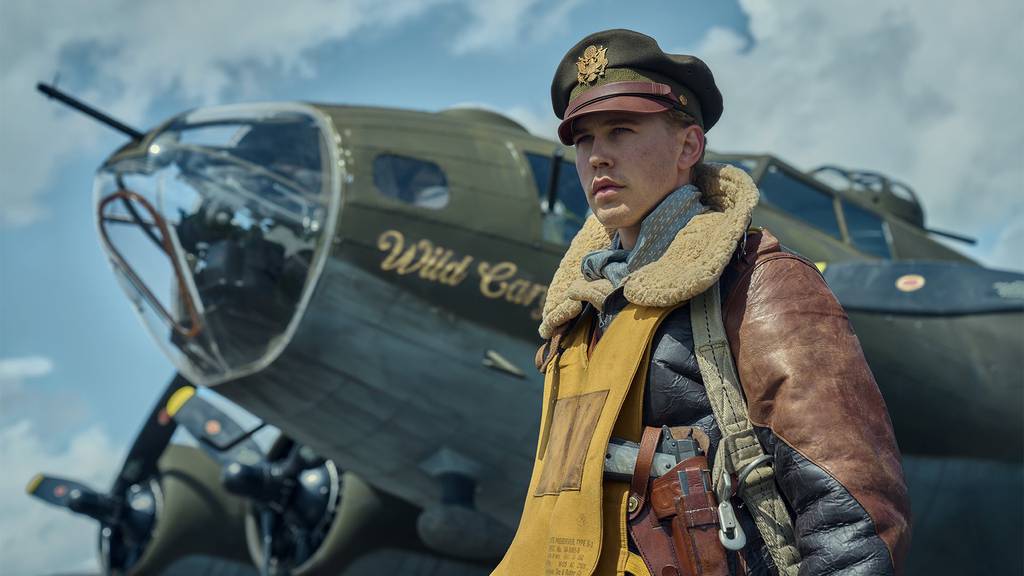The image depicts a young World War II military pilot, dressed in a dark brown and black leather bomber jacket with a wool shearling collar, and a yellow protective vest. He sports a green military-style hat with a brown brim and a gold badge, alongside a blue scarf and a holstered pistol with a brown holster. The pilot stands in front of a vintage Army khaki-green fighter jet, likely from the World War II era, adorned with black propellers and gun turrets both at the front and back. The plane has partially visible inscriptions in yellow that read "Wilde" and "CAR," though the full text is not discernible. The setting has a clear blue sky with scattered clouds, emphasizing the historical and military ambiance of the scene.